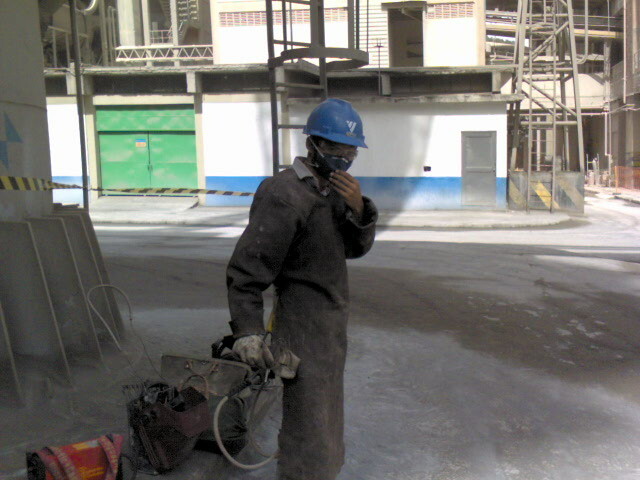This detailed photograph captures a construction worker standing on a dusty construction site. The worker is dressed in a gray, dust-covered uniform and wears a distinctive blue hard hat featuring a white triangle design on the front. A black face mask and goggles obscure much of his face, and his right hand is raised, touching the mask as he glances back at the camera.

Surrounding the worker are various equipment and tools; to his left lies a red tool bag and additional tools scattered on a bench. A nearby object, possibly a lamp, stands out with its red and yellow coloring.

The background reveals a bustling construction scene. A blue and white building, accentuated with a blue stripe along the bottom, stands prominently. This building, surrounded by scaffolding, appears to be a significant ongoing project. A gray building to the left bears a nuclear symbol, adding an intriguing detail to the scene. Additionally, green doors, multiple ladders, and climbing equipment can be seen around the site. A yellow and black rope cordons off an area where a car is parked, and caution tape stretches across the street, emphasizing the active and safety-conscious environment of the construction zone.